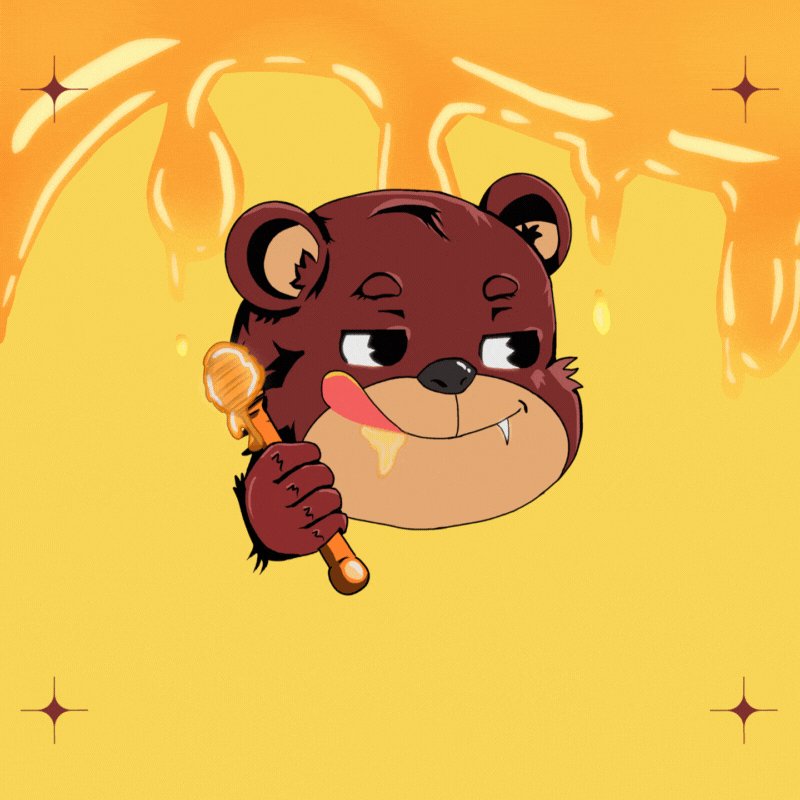This image depicts a vibrant cartoon drawing of a bear's face set against a dynamic background. At the top of the image, a rich amber color resembling glistening honey drips down into a yellow background, creating a striking effect. The bear's face, predominantly dark brown with lighter brown around its mouth and ears, is positioned in the center, looking to the right. The bear's black-and-white eyes add a touch of vivid contrast. The inside of its ears is imbued with a peach color, and its nose is black. From the left side of its tan-colored mouth, a pink tongue extends outward with a glossy drop resembling honey hanging from it. Additionally, the bear's right paw is visible, clutching a honey dipper that is also dripping with honey. Each corner of the image features a brown plus sign, adding a sense of balance to the composition. Overall, the image is a playful and richly detailed representation that evokes the charm of classic bear illustrations, possibly inspired by the Berenstain Bears.